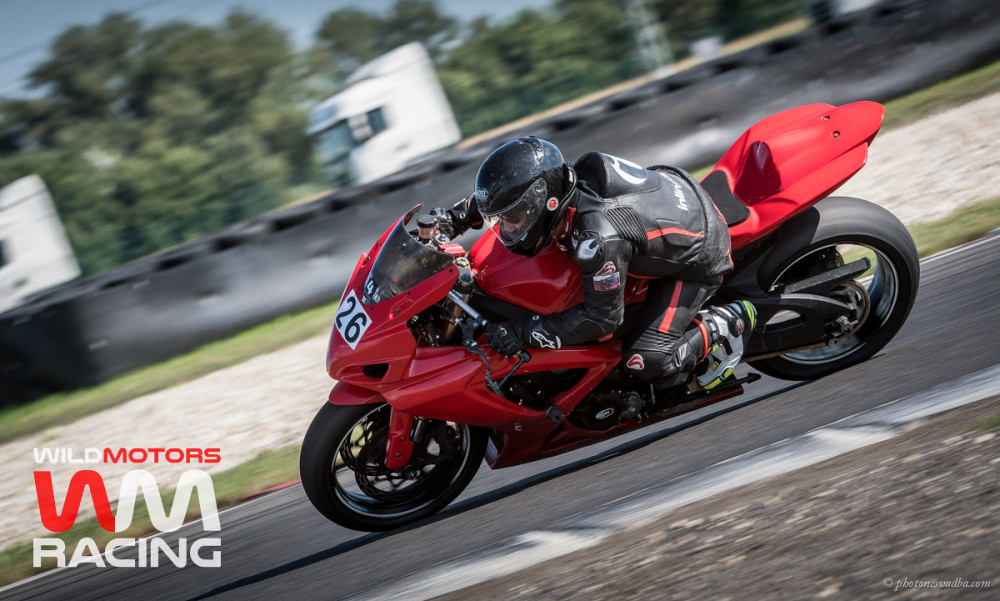This is a horizontally aligned rectangular picture depicting a high-speed motorcycle race. Centered in the image is a red sports bike, adorned with the number 26 in black letters against a white square background. The motorcyclist, tilting to the left, is clad in a black helmet and a black leather outfit with red stripes and some unreadable white text on his back. In the lower left-hand corner, the text "Wild Motors WM Racing" is displayed, with "Wild" in white, "Motors" in red, and "WM" in alternating red and white letters, followed by "Racing" in white.

The background features a blur of green-leaved trees and a hint of a blue sky. The upper left-hand corner of the image reveals the fronts of some white trucks. Behind the motorcyclist, a strip of grass and a black safety wall, possibly made of tarp, is visible. In the foreground, the road is partially visible in the lower right-hand corner, marked with a tiny copyright symbol and an unreadable name, along with some dirt and rocks leading into the track.